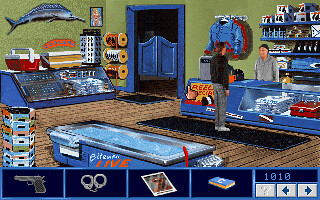This still image, appearing to be taken from a slightly pixelated video game, depicts a bustling store scene. The shop's walls are green with a blue-framed doorway, creating a welcoming yet rustic atmosphere. The wooden plank floor adds to the quaint charm of the setting, while various displays, cabinets, and shelves line the room, showcasing an array of items. On the left side of the room, a large mounted marlin or swordfish grabs attention, enhancing the decor with a maritime touch.

Dominating the scene are two Caucasian male characters: one behind the counter, who seems to be the shopkeeper, and another in front of the counter, likely a customer. The shopkeeper's area is cluttered with boxes and shelves overflowing with goods, including clothing items in blue and red colors hanging on the wall. Numerous spools, potentially of thread, and rotating racks filled with different products dot the background, along with what appears to be a large refrigeration case embedded in the floor.

At the bottom of the image, a grid interface typical of video games is visible, displaying various icons: a gun, handcuffs, a photograph, a book, possibly some money, and numerical values accompanied by directional arrows, indicating in-game information and options.